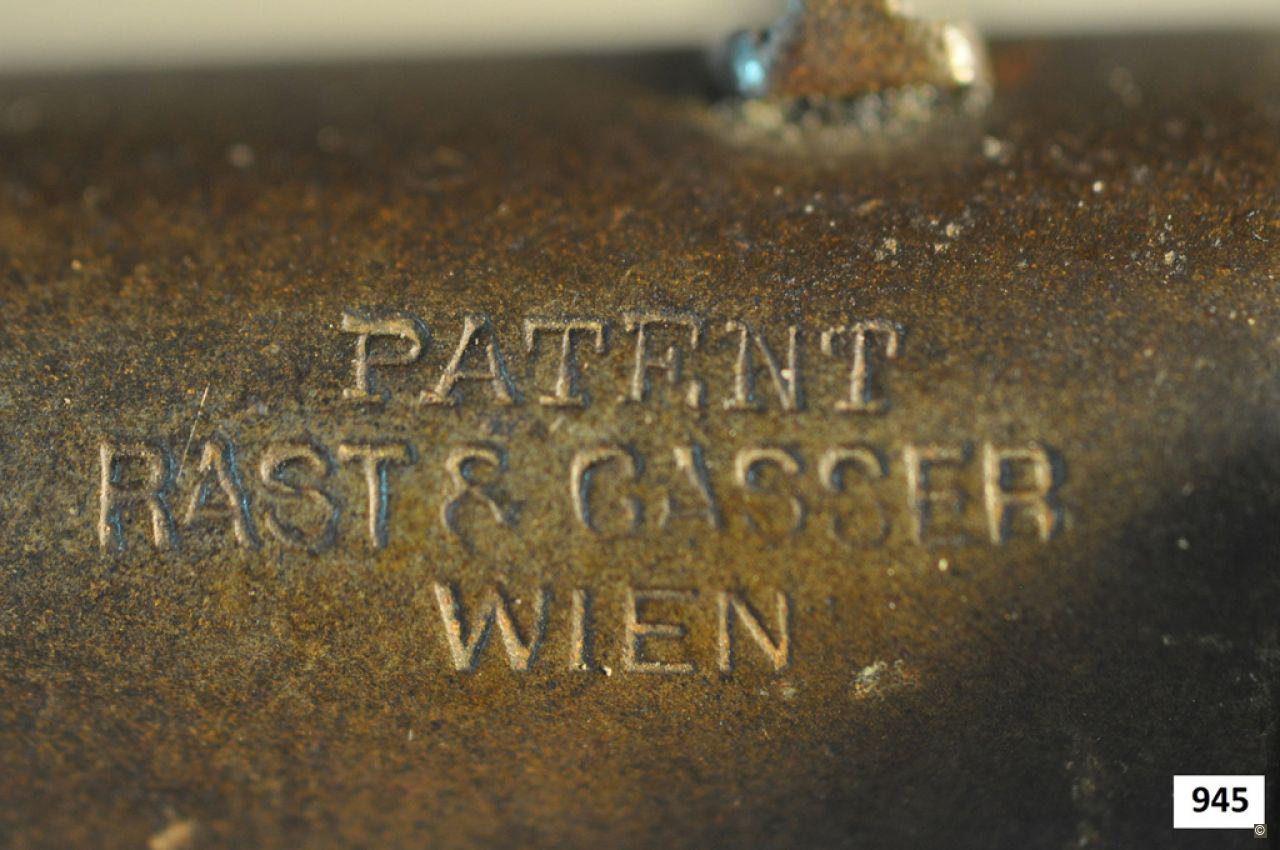This detailed color photograph showcases a very close-up view of a rusted metal surface, likely a piece of machinery. The metal, which has a burnished brass or pewter-like appearance, features raised, embossed lettering. The print starts at the top with the word "patent," followed by "Rast and Gasser," and "Wien" (W-I-E-N) below. In the lower right corner, "number 945" is clearly visible within a white box with black text. The image also reveals notable signs of wear and corrosion: there's a blurry, reddish-brown area at the top where a small chunk of the metal seems to be missing, suggesting rust damage. Scattered black rust and tiny white specks further highlight the surface's aged and oxidized condition.